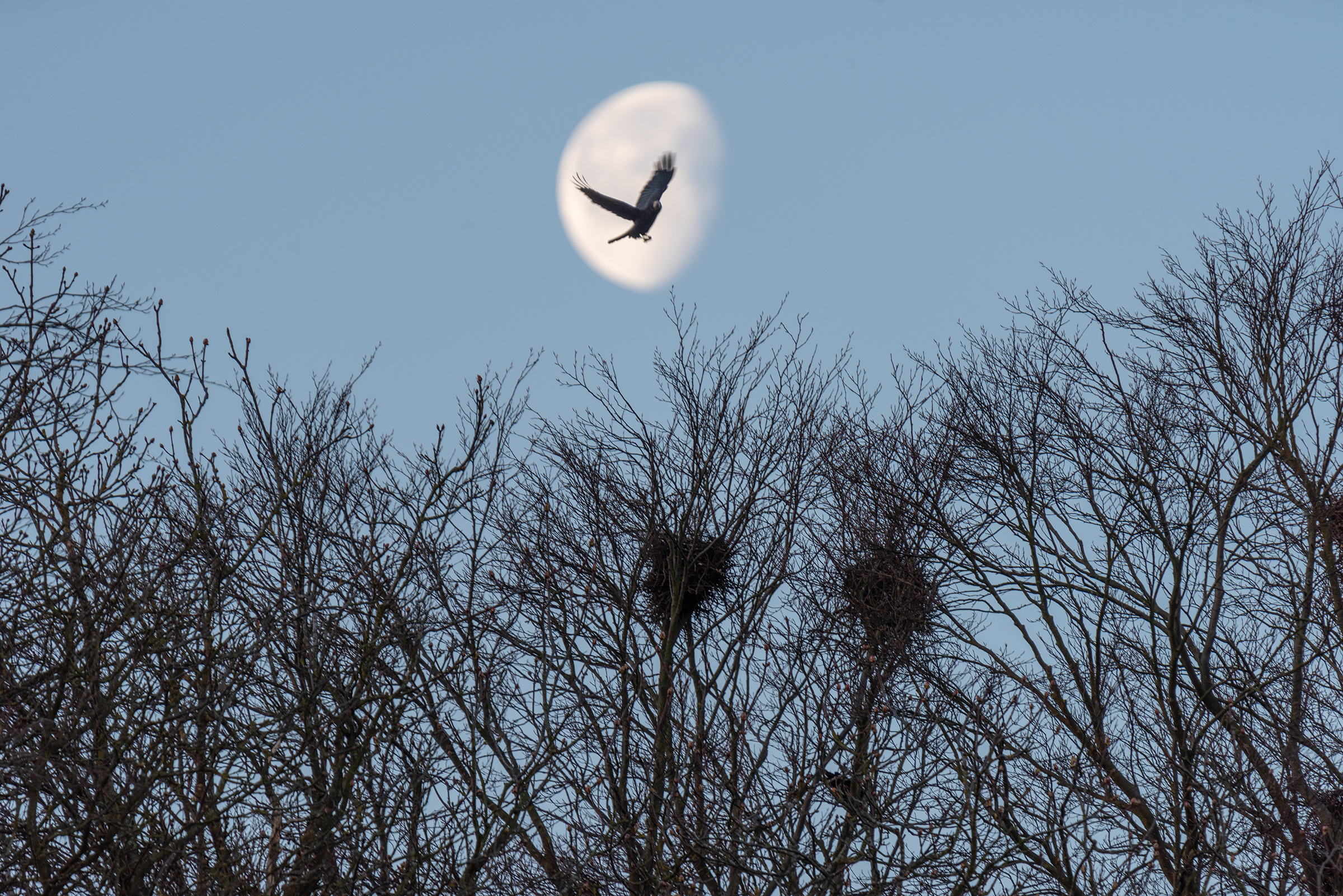In this photograph, a sizeable bird, likely a hawk or eagle, soars through the sky. The image, taken from a distance, captures both the bird and its surroundings, creating a sense of vastness. The bird's wings are fully extended, and it appears to fly directly over a prominent moon, which occupies the center of the scene. The sky is a grayish-blue, adding a serene backdrop to the image. Below the bird, there are tall, leafless trees with bare branches intertwined like a web of twigs. The trees, devoid of green leaves, have a few patches of brown or orange foliage that almost blend with the branches. Noticeably, two of these central trees contain large nests made of sticks near their tops. The overall composition of the photo, with the bird in majestic flight over the moon against the stark branches of the trees, evokes a sense of calm and natural beauty.